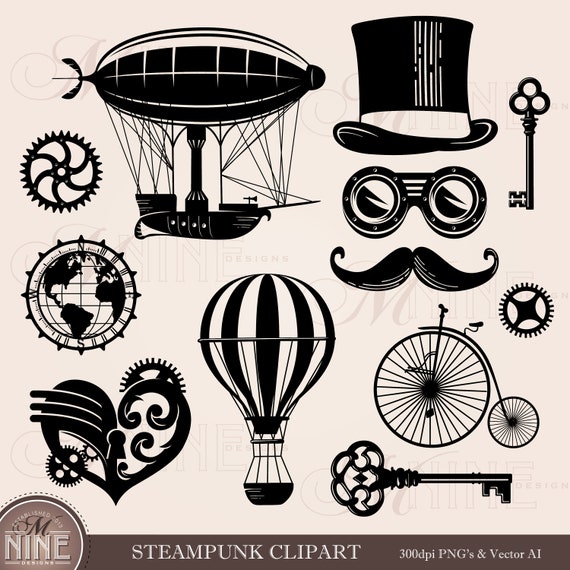The image is a square, vintage-style illustration, possibly from a book or displayed on a computer screen, measuring approximately four inches by four inches. The background is a light pinkish-brown tone. It features a collection of detailed black and white steampunk clipart images arranged in a grid format. At the top left is a hot air balloon tethered to a ship with multiple cords. Next to it is an all-black gear cog. Below these is a top hat adorned with goggles and a mustache underneath. Nearby is a classic skeleton key and a globe encircled by compass points. Further down is a stylized heart embedded with gears and cogs. Adjacent is an old-fashioned penny-farthing bicycle, characterized by a large front wheel and a small rear wheel. Lastly, another hot air balloon with a hanging basket is depicted, along with a smaller cog and another key. 

At the bottom, there's a slender light brown banner with a circular emblem stating "Established 2013," followed by the text "Nine Designs." To the right, the banner reads "Steampunk Clipart, 300 DPI PNGs and Vector AI."